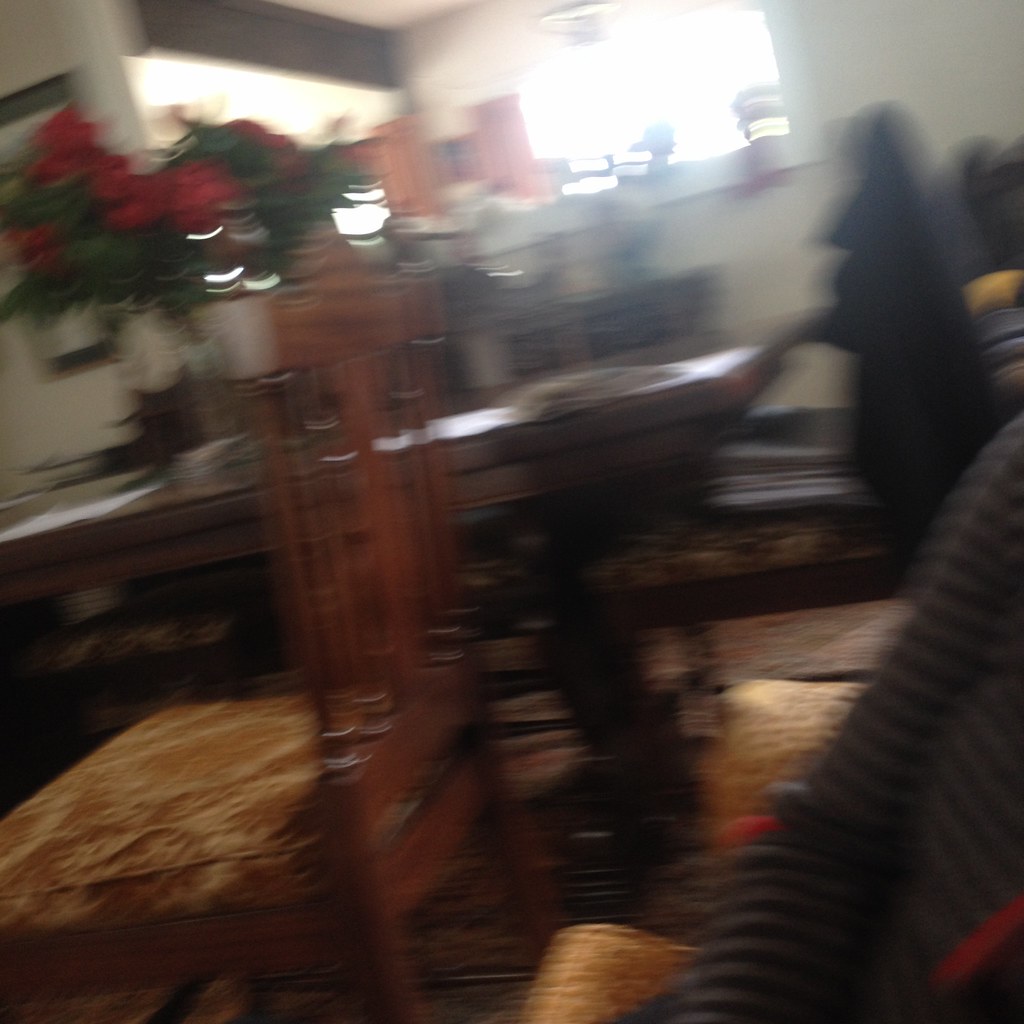In this blurred and tilted image of a private home, sunlight streams through the open curtains of a window in the background, illuminating the room with a warm glow. In the center, a long, dark brown walnut dining table is adorned with white placemats and an arrangement of red flowers, possibly poinsettias, though it is unclear whether they are in a vase. Surrounding the table are several brown wooden chairs, with one prominently positioned in the forefront featuring a gold or damask-covered cushion. A picture frame hangs on the left wall, though its details are obscured by the blur. To the right, there appears to be a black, ribbed vacuum cleaner hose. Beyond the dining setup, there is a credenza topped with a few decorations and a lower cabinet, adding depth to the scene. Despite the lack of clarity, the interplay of furniture and sunlight suggests a cozy, lived-in space.